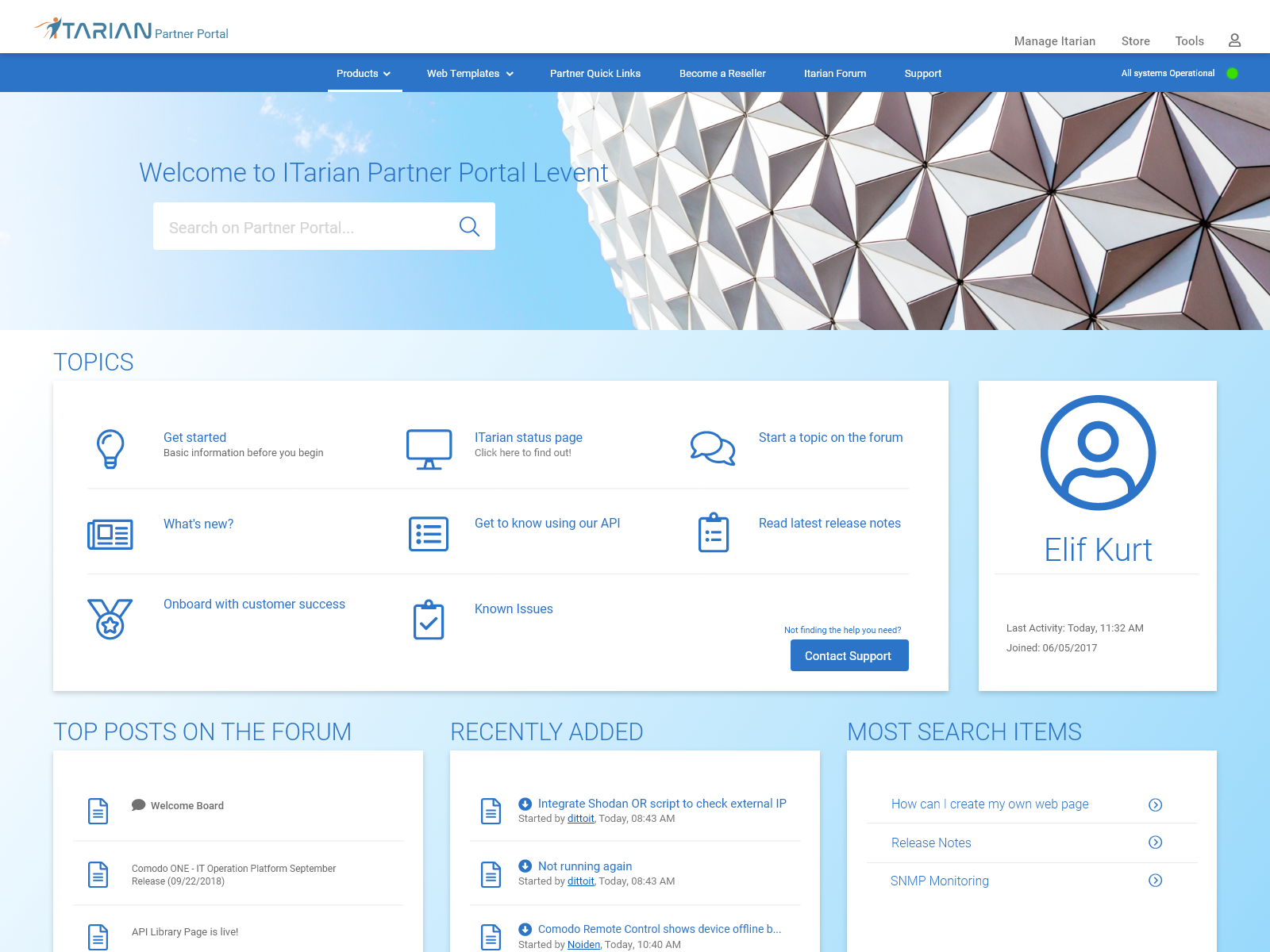This is an image of the Terrian Partner Portal interface. In the upper left-hand corner, the site title "Terrian Partner Portal" is displayed in vivid blue letters. The color scheme throughout the page is a clean blue and white.

On the left side of the interface, there are navigational options listed in white text: Products, Web Templates, Partner Quick Links, Become a Reseller, Terrian Forum, and Support. On the right-hand side of the page, the status "All Systems Operational" is shown, also in white text. Above this status message, there is a section labeled "Manage," featuring the I Terrian Store, Tools, and a small person icon, all in black lettering.

Beneath these elements, a circle of white diamonds is depicted. Below this decorative element, there is a search bar with the placeholder text "Search on Partner Portal." Directly above the search bar, in bold blue letters, it says "Welcome to I Terrian Partner Portal Events," situated against a light blue background with a white sky design.

Under this header, there is a list of topics presented for user navigation, including: "Get Started," "What's New," "On Board with Customer Success," "Known Issues," "Get to Know," "Using our API," "I Terrian Status Page," "Start a Topic on the Forum," "Read Latest Release Notes," and "Contact Support."

In the user profile section, it shows that the logged-in user is Elif Kurt. The profile details note that Elif Kurt's last activity was today at 11:32 AM, and their membership began on June 5, 2017.

Further down, the portal features sections for "Top Posts on the Forum," "Recently Added Items," and "Most Searched Items," providing users with easy access to important content and updates.